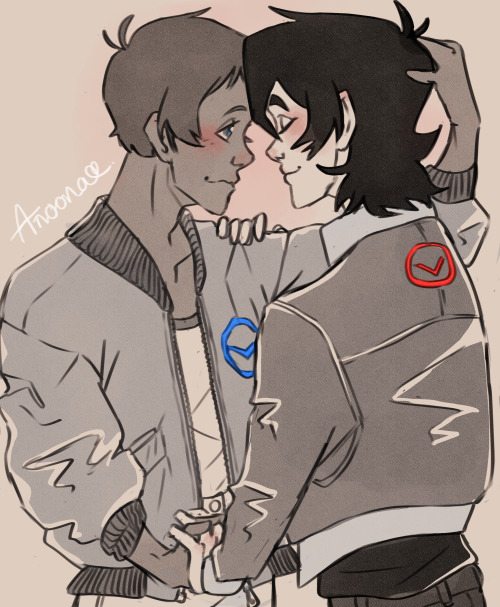The image depicts an anime-style, grayscale drawing of two male characters engaging in an intimate pose, emphasizing their emotional connection. Positioned against a medium-gray, vertically-aligned rectangular background, these sketched figures are shown from the top of their heads down to their waists. The character on the left has darker skin and short brown hair, while the character on the right has lighter skin and slightly longer black hair. They are leaning against each other with their foreheads touching, seemingly about to kiss. The left character's right hand clasps the right character's left hand in the foreground, while his left hand rests on the right character's shoulder. The right character's right hand is gently placed on the back of the left character's head. Both are wearing brown varsity-style jackets, with the left character’s featuring a blue circular emblem with a 'V' on the ribbed collar, and the right character's similar emblem, in red, located on the upper back. Notably, the left character's eye is open, gazing warmly at the other, whose eyes are closed. The artist's signature, reading "ANUNE", is inscribed in white cursive on the upper left side of the image.